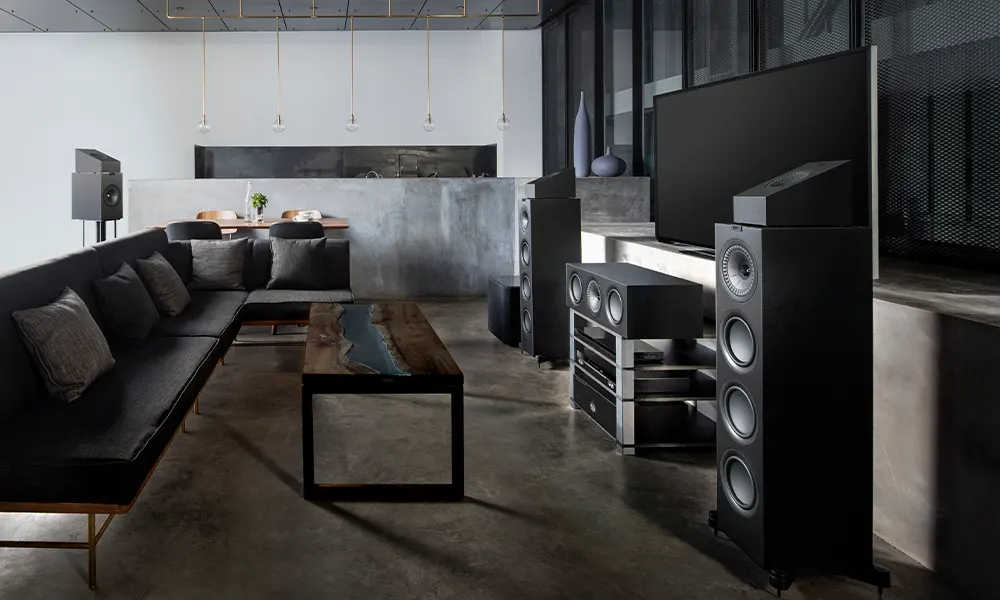This detailed photograph captures a modern living room with a sophisticated home theater system in a landscape layout. Dominating the left half of the image is an L-shaped black sofa adorned with gray pillows, and in front of it, a unique coffee table featuring three bars—brown on the outer sides and blue in the middle. At the center of the room stands a black subwoofer with three ports, flanked by two towering speakers on either side of a large, flat-screen TV. Each of these speakers boasts four woofers, creating an immersive audio experience. Behind the sofa is an additional speaker, suggesting a five-point home theater setup.

The background features a striking design with a half silver wall, above which are gold pendant lights hanging from a black ceiling. The wall behind the entertainment system contrasts with a black upper section and a gray-silver charcoal lower section. The brown, shiny concrete floor adds a sleek touch, complementing the room's overall modernistic and monochromatic aesthetic.